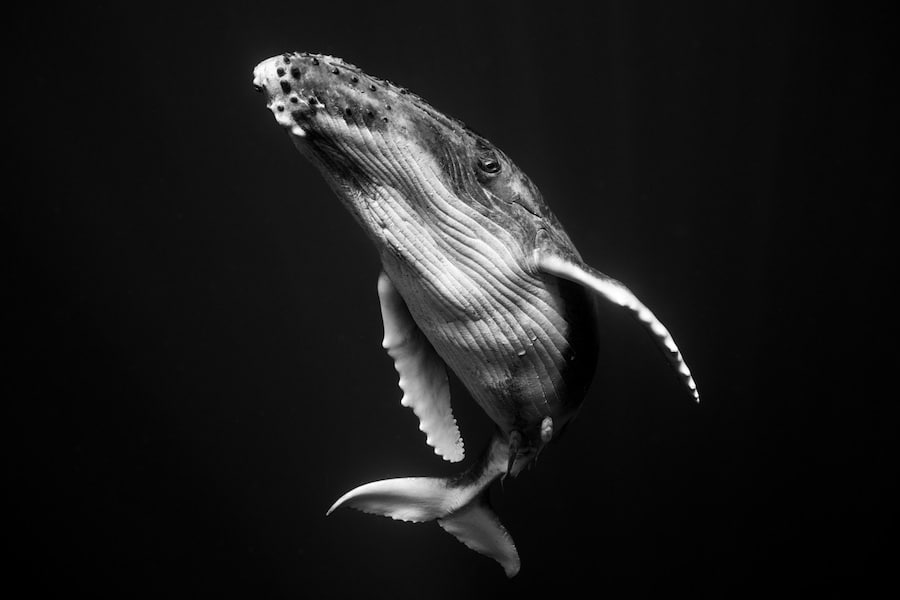This stark, black-and-white image features a highly detailed depiction of a whale—likely a humpback—suspended against a pure black background. The whale is shown from an upward angle, allowing close examination of its snout, fins, and underbelly. The whale’s eye is visible, highlighting its lifelike presence. The underbelly displays long, grooved wrinkles, while the top is darker, with what appears to be bumpy or rocky textures on the snout. There is some ambiguity regarding the background's nature and whether the image is a photograph or a meticulously crafted AI creation, yet the whale remains the singular, striking subject of the composition.